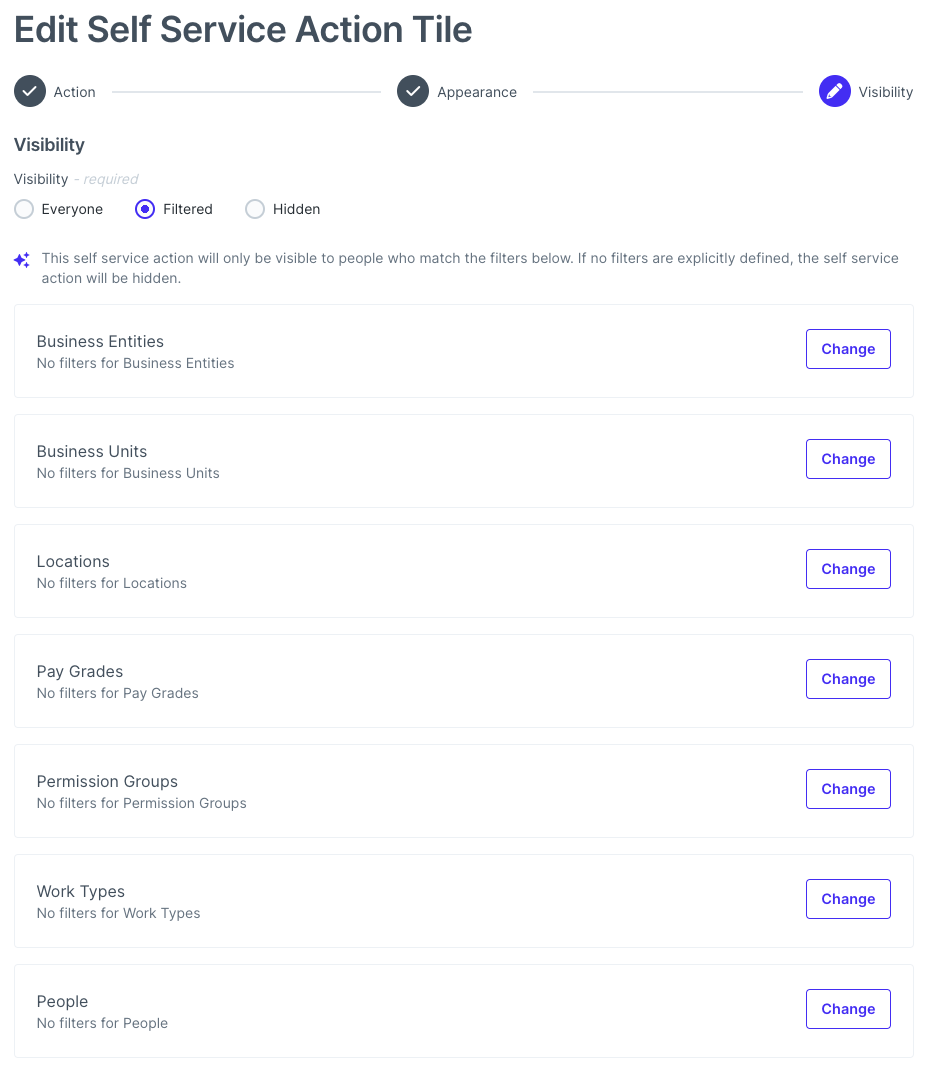The image displays a user interface section for editing a "Self-Service Action Tile." The layout is structured and visually categorized as follows:

- **Title**: "Edit Self-Service Action Tile" in bold black letters at the top.
- **Status Indicators**:
  - On the left: A black circle with a white check mark labeled "Action."
  - In the middle: Another black circle with a white check mark labeled "Appearance."
  - On the right: A blue circle containing a white microphone icon labeled "Visibility."

Below the "Visibility" section, three distinct status options are listed side by side:
  - A white circle, labeled "Everyone."
  - A blue-outlined circle with a blue dot at the center, labeled "Filtered."
  - An empty circle, labeled "Hidden."

- **Categories**:
  - Multiple vertically aligned rectangles, each representing a different category. Categories are listed in bold black text on the left:
    1. Business Entities
    2. Business Units
    3. Locations
    4. Pay Grades
    5. Permission Groups
    6. Work Types
    7. People

- **Action Buttons**:
  - Each category rectangle has a corresponding rectangular blue-outlined button on the right side, each labeled "Change."

This detailed layout clearly categorizes different elements of the interface, providing distinct sections for easier navigation and specific action-taking opportunities.